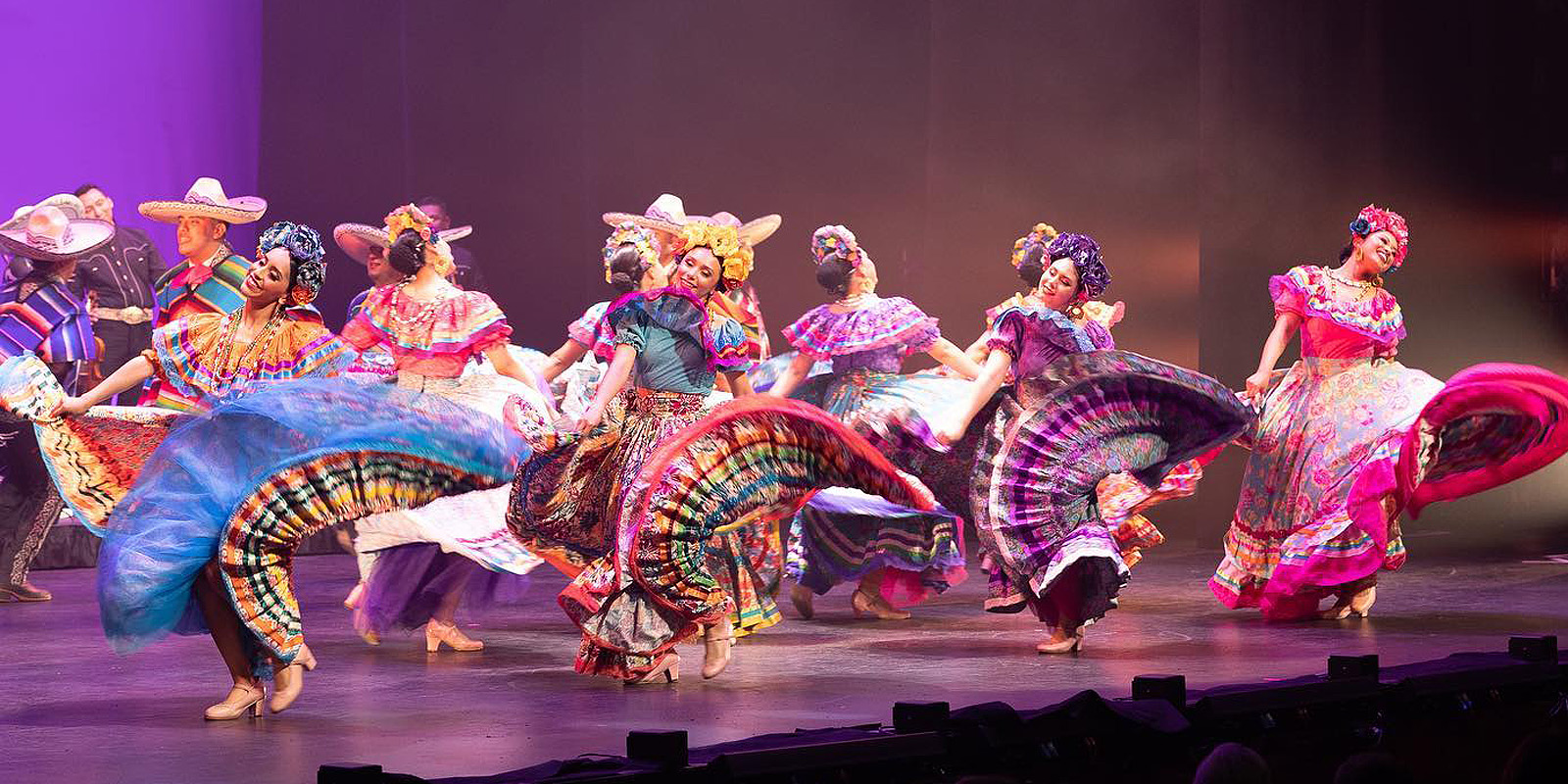In this photograph, a dynamic scene unfolds on stage featuring approximately 10 to 15 dancers, primarily women, clad in vividly colorful traditional South American attire. The stage, set in a landscape-oriented rectangular frame, is awash with purple hues from the lighting, creating a vibrant contrast against the dark floor. Predominantly in the foreground are women adorned in long, multicolored dresses of blues, purples, pinks, yellows, greens, and reds, complemented by swirling skirts in mid-motion, indicating an active dance.

The women also wear elaborate headpieces, including flower crowns, which add to the festival of colors. In the background stand the male dancers, who are attired in equally colorful ponchos and sombreros, which suggest traditional Mexican influence. Their presence offsets the scene with a cultural richness, as they sway to the rhythm in their brown boots. The background amplifies the performance's liveliness with a completely purple wall on the far left, adding depth to the photo. Smiles and exuberance define the faces of these South American dancers, resonating with the joy and energy of their performance.